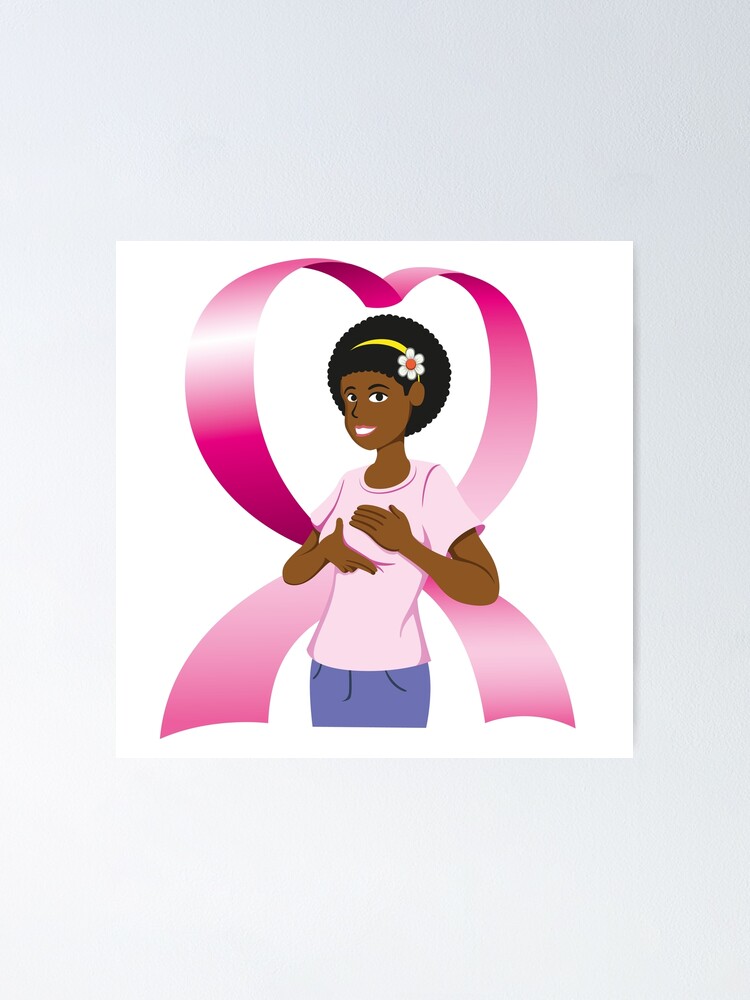This is a detailed, color computer-generated illustration of an African American woman conducting a self-breast exam. She is shown smiling directly at the viewer, revealing her teeth, while delicately holding her breasts with both hands over a pink short-sleeved shirt. The woman has short-cropped hair adorned with a yellow headband featuring a white daisy. She exudes a cheerful demeanor, emphasized by the bright and lively colors in the image. She is a thin woman and appears to be wearing a purple skirt or pants, although part of her lower body is cut off in the illustration.

In the background, a large pink ribbon, symbolic of breast cancer awareness, prominently curls in the shape of a heart, with its top extending over her head. There is no text in the image explaining the context, but it evidently aims to promote Breast Cancer Awareness Month or Breast Exam Awareness through its vivid and uplifting depictions.